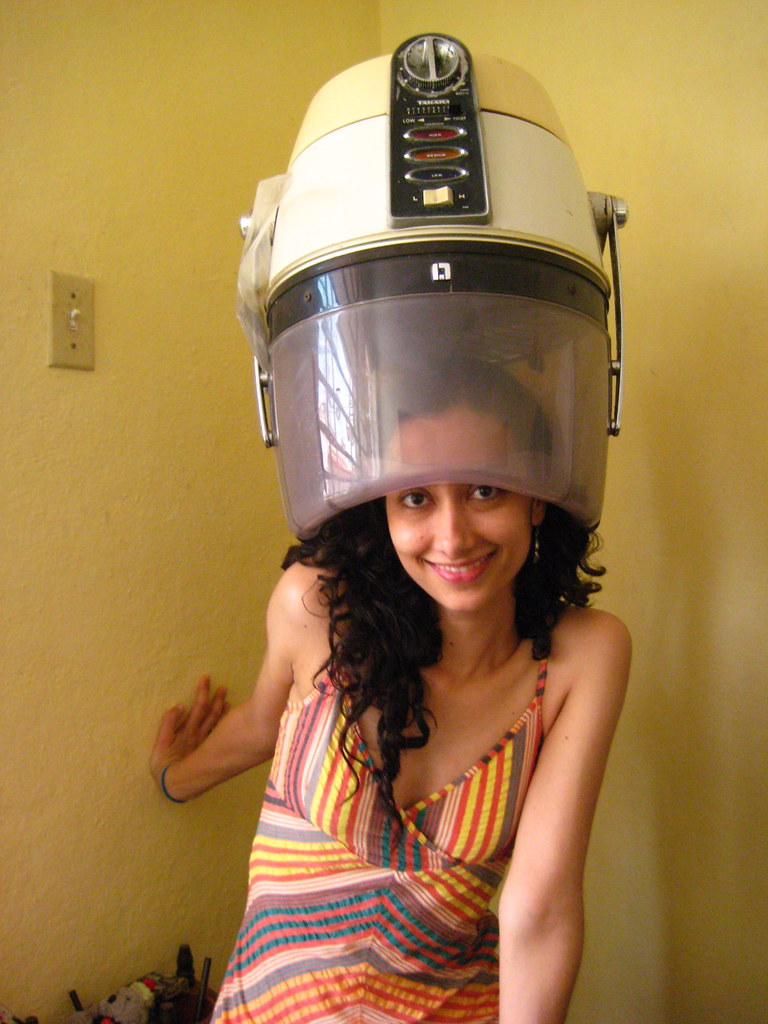The photograph shows a young woman with long, dark, curly hair smiling directly at the camera. She is wearing a vibrant sundress featuring multi-colored stripes in shades of orange, yellow, blue, green, brown, and white. The dress has an off-shoulder design, exposing her right shoulder. She stands in the corner of a room with yellow walls, one of her hands placed on the wall at an awkward angle, while the other is positioned behind her.

Notably, an old-fashioned beauty salon hairdryer hovers above her head. The hairdryer is an outdated model, identifiable by its oval-shaped buttons and a little white plastic on-and-off switch at the front. Part of the hairdryer is made of slightly hazy clear plastic, covering the top of her head and partially obscuring her forehead. Above her right hand is a light switch, while some indistinct tools or items can be seen on the floor nearby, making it hard to determine if she is sitting or crouching. The overall scene exudes a playful, nostalgic charm, with the woman joyfully posing in this surreal setup.